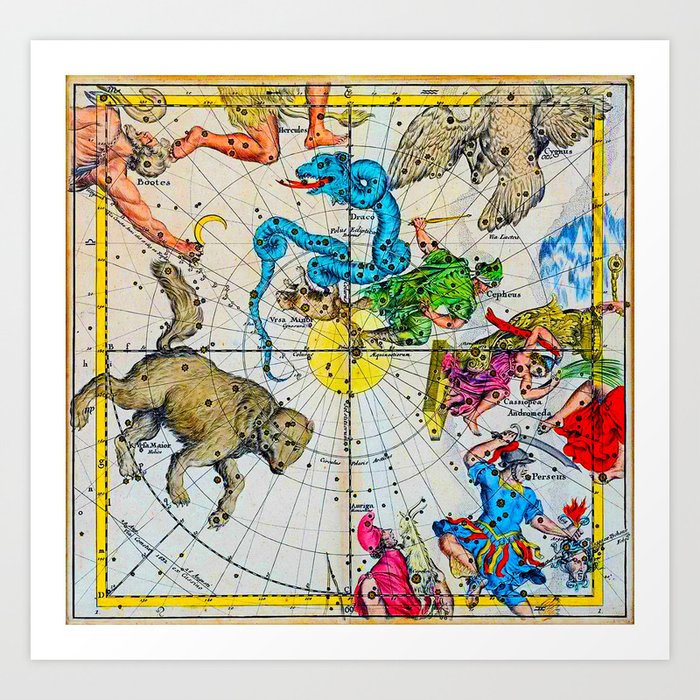This detailed digital star map evokes a vintage aesthetic with its layered beige and yellow translucent borders. Featuring a grid layout, it displays representations of constellations and Greek gods, vividly illustrated across the celestial landscape. On the top left, an older bearded man named Bhutia holds a moon, while to his right, images continue: feet, a feathered animal, a jester on its side, and a warrior named Perseus in blue with yellow and red tassels, wielding a sword overhead and holding Medusa’s head. Adjacent to him, a person in hot pink, named Aurigon, carries a goat on their back. The final image on this row depicts a bear labeled Maior. 

Centrally located is a green-hued figure with a sword on his hip, asserted to be another deity. Beside him coils a blue serpent with a red tongue named Draco. The yellow-centered map radiates with circles and lines reminiscent of coordinates, mapping out constellations and dotted with stars. Names such as Perseus, Cassiopeia, Andromeda, Cepheus, and Cygnus are inscribed, though not all legible, each identified with their respective icons: Cassiopeia as a pink-clad woman, and Cygnus as a bird. This star map, enriched with detailed annotations and mythical figures, serves as an illustrative guide to the constellations.